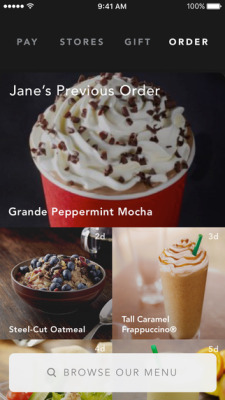The image appears to be a screenshot from a mobile application displaying specialty coffee drinks. The background is black, with a status bar at the top: five white dots on the left, the Wi-Fi icon in the middle, and '9:41 AM' along with a fully charged battery icon to the right. Below the status bar, a menu in bright white font reads: 'Pay', 'Stores', 'Gift', 'Order', and 'Orders'.

Underneath the menu, there are images and descriptions of specific items. The first item is labeled as 'Jane's Previous Order', featuring a picture of a Grande Peppermint Mocha in a festive red cup with a white rim. The mocha is topped with white whipped cream and garnished with chocolate sprinkles, with the mocha's brown liquid visible beneath.

Adjacent to this is an image of 'Steel Cut Oatmeal'. The oatmeal is served in a brown bowl, placed on a brown table, topped with blueberries and the oatmeal's natural brown hue is visible.

To the right, there's a picture of a 'Tall Caramel Frappuccino'. It is served in a transparent glass filled with a brown liquid, topped with white whipped cream and a drizzle of brown caramel. A green straw is inserted into the drink, which is positioned against a lighter brown table, with a white glass in the background.

On the lower part of the image, there is a search bar enclosed in a white square box, featuring a grey magnifying glass icon accompanied by the words 'Browser menu' in grey font.